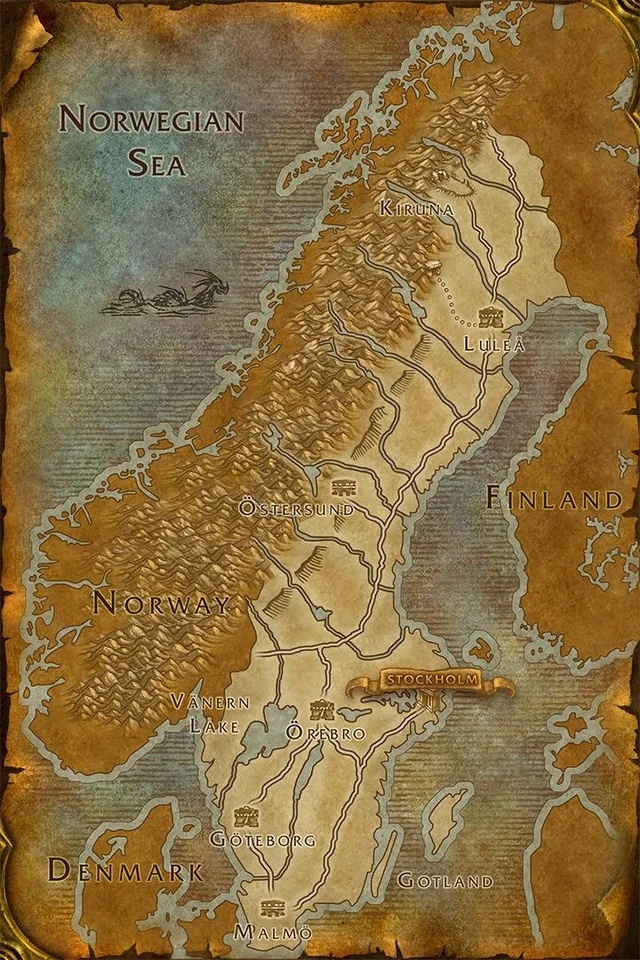This detailed map, rendered in a vintage, manila and tan color palette, prominently features Scandinavia, including Norway, Sweden, Finland, and Denmark. The Norwegian Sea, highlighted in blue with an illustrated dragon, occupies the top left corner of the map. Distinct geographical features include a large mountain range stretching across Norway, with horizontal lines representing the water. Key cities labeled on the map include Stockholm, featured in a central golden banner, Gothenburg, Malmö, and the island of Gotland in Sweden, as well as Östersund, Bergen, Luleå, and Kørnen. Denmark is positioned at the bottom left, and Finland is towards the center-right. The map's text is in fine print, giving it an arctic feeling, with Norwegian and Scandinavian countries outlined in black and highlighted in white. This topographical map of Scandinavia showcases its cities and geographic features in a detailed and historic style.